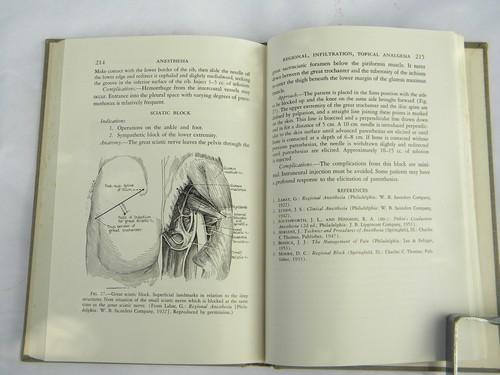The image depicts an open medical book, specifically displaying pages 224 and 225, placed on a light gray or white marble table. The book’s pages are light tan in color with black and white sketches, predominantly featuring anatomical drawings. The left page showcases an image of muscles, likely focused on the sciatic region of the human body, accompanied by two paragraphs of text. The anatomical illustration appears detailed, depicting muscles and tissues in a monochrome, sketch-like style. On the right page, there are several paragraphs of text and a list of references. Additionally, there's a depiction of a tool in the bottom right-hand corner, possibly a medical instrument with a distinctive L-shape. The book itself has a dark gray cover and binding, adding a contrast to its lighter pages. The image is blurry, making precise text difficult to read, but it’s clear the focus remains on the detailed anatomical illustrations and associated descriptions.